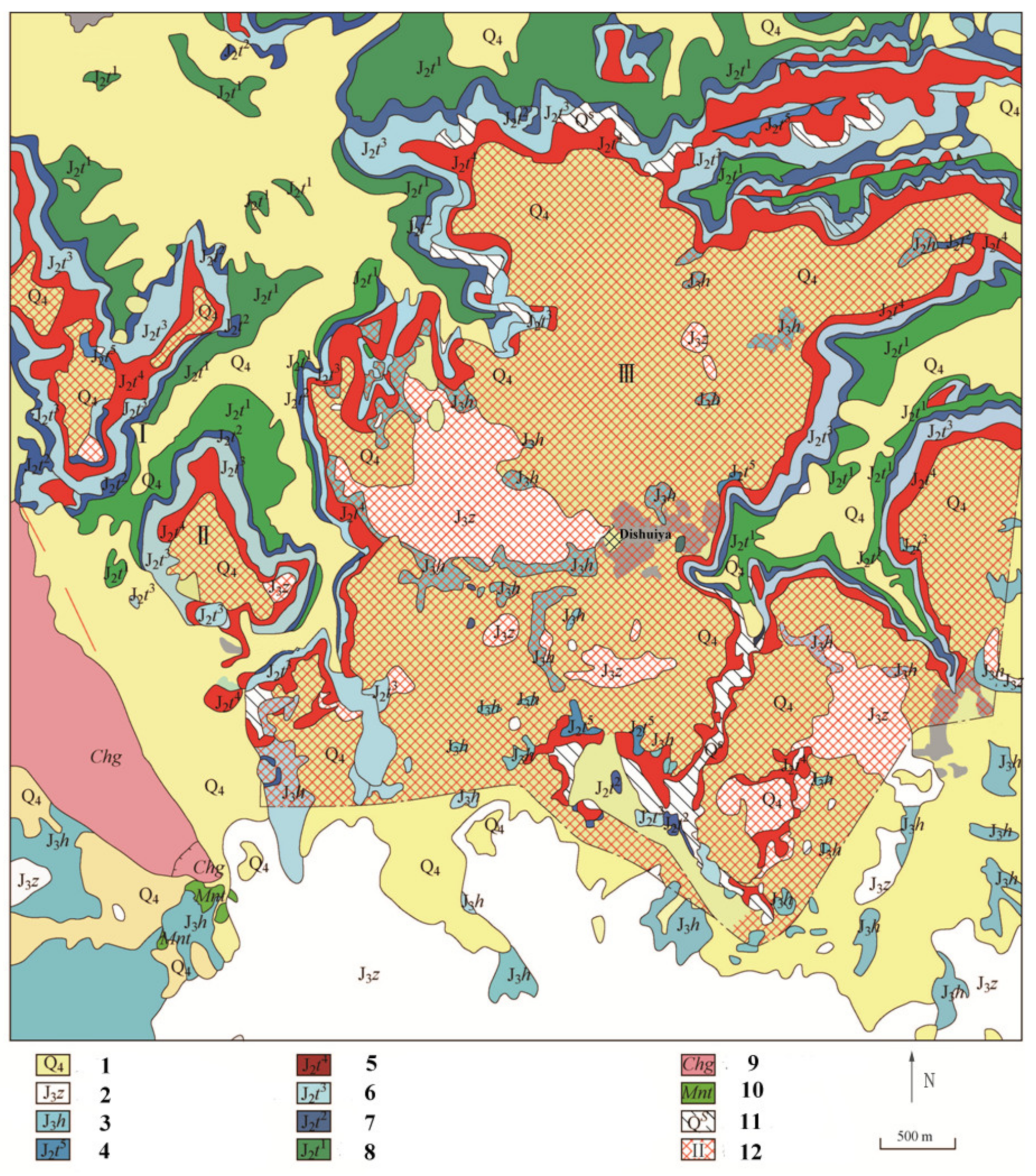The image depicts a detailed aerial view of a map, featuring a variety of colors and outlined regions that correspond to different areas or countries. Each area is uniquely colored according to a legend located at the bottom of the map. The map uses a yellow background and has multiple lines crisscrossing it, making it somewhat difficult to read. Light blue sections likely denote water, while dark green regions may indicate mountain areas. Large areas are shaded in light brown, possibly representing the ground or land.

In the middle of the map, there's an orange section with a white checkerboard pattern, labeled "Q4." Surrounding it are various regions such as a red area, a light blue section marked "J2R," a green section labeled "J23," and a yellow section also labeled "Q4." These colors and labels are dispersed throughout the map, indicating different sections or zones.

The legend at the bottom provides a key to the colors, numbered 1 through 12, with each number corresponding to a colored rectangle. The colors range from yellow (number 1) and white (number 2) to dark blue (number 7) and a crosshatched red line pattern (number 12). The legend helps to identify the regions on the map above. Additionally, the bottom right corner features an arrow labeled "N," pointing north, and a scale bar indicating 500 meters per inch.

Overall, this highly detailed map serves as an intricate guide, possibly for geopolitical or geographical purposes, with a complex layering of colors, labels, and regions.